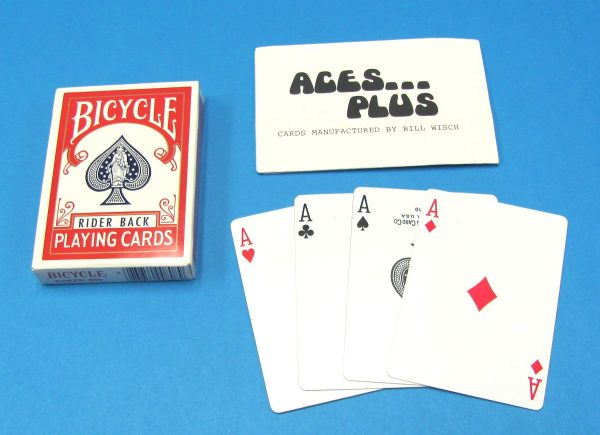This color photograph, taken in landscape orientation, features an array of playing cards and related objects meticulously arranged on a solid blue surface. On the left side of the image lies a Bicycle Riderback Playing Cards box. The front of the pack, facing the viewer, displays a red and white design, prominently featuring a blue spade symbol in the center, with "Bicycle" written at the top and "Playing Cards" at the bottom in large white letters. Notably, the side of the box includes a scanning barcode and an upside-down heart motif. 

To the bottom right of the image, four aces—each from a different suit—are fanned out in a row. From left to right, they are the Ace of Hearts, Ace of Clubs, Ace of Spades, and Ace of Diamonds. Positioned just above these aces is a white card, bearing the text "Aces... Plus" in bold black letters, with the additional notation "Cards manufactured by Billwish" in smaller black print underneath.

The vivid colors in the scene, including the blue of the background, and the varied hues of the cards—blue, white, black, red, and gray—combine to give the image a dynamic yet orderly appearance. This setting evokes a sense of anticipation, as if someone is about to engage in a game of cards.